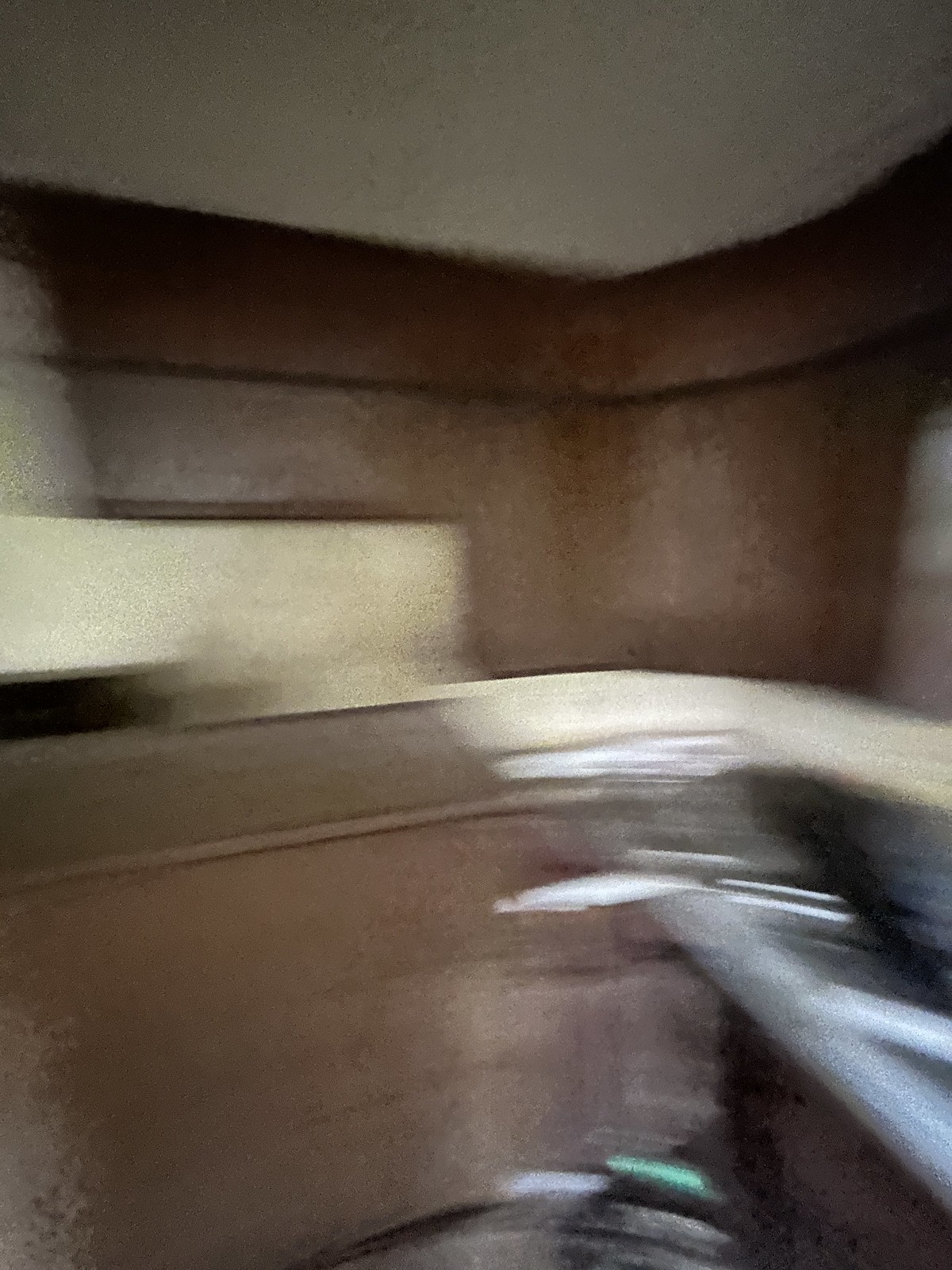This photograph captures a blurry and out-of-focus interior of a room, providing a somewhat chaotic yet intriguing view. The image is dimly lit, casting a subdued ambiance throughout. The central focus appears to be the corner of the room where two walls meet, both adorned with a dark brown design element that runs along the ceiling and descends along the wall and across a countertop before rising back up to the ceiling. The walls themselves are primarily cream or white with a yellowish tint, possibly due to dirt or aging. The ceiling is white, contrasting with the darker tones of the woodwork. 

In the lower right-hand corner, there is an indistinct gray and silver object that suggests the presence of something metallic, perhaps resembling a dental chair. Alongside it, blurry green objects hint at some form of vegetation or decor near a countertop that features a blend of light and dark gray hues. Additionally, the blurred black outlines on both the left and right sides of the image add to the confusion, making it difficult to clearly identify these elements. Light reflections appear from an undefined source, enhancing the sense of depth despite the image's overall fuzziness.